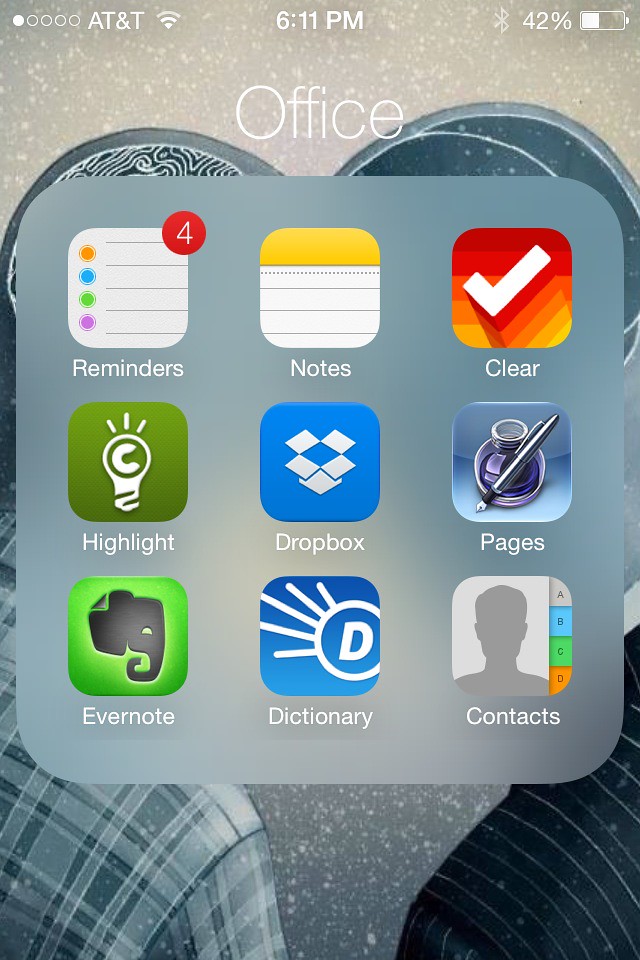The photograph captures a close-up of someone's smartphone screen. In the top left-hand corner, the phone displays poor reception with one out of five bars, indicates it is connected to AT&T, and shows an active Wi-Fi connection. The time displayed is 6:11 p.m. On the top right corner, the phone’s Bluetooth is enabled, and the battery level is at 42%.

The main focus of the photograph is a folder titled "Office" open on the screen, showcasing various apps inside. The apps visible within the folder include:
- Reminders (with a notification badge indicating four pending reminders)
- Notes
- Clear
- Pages
- Dropbox
- Highlight
- Evernote
- Dictionary
- Contacts

Behind the opened folder, the background is partially visible, showing what appears to be the shoulders of two individuals. The details of the background are obscured by the folder interface, but the presence of people is noticeable. The overall image provides a detailed glimpse into the user’s phone setup and current screen content, blending both functionality and incomplete background visibility.